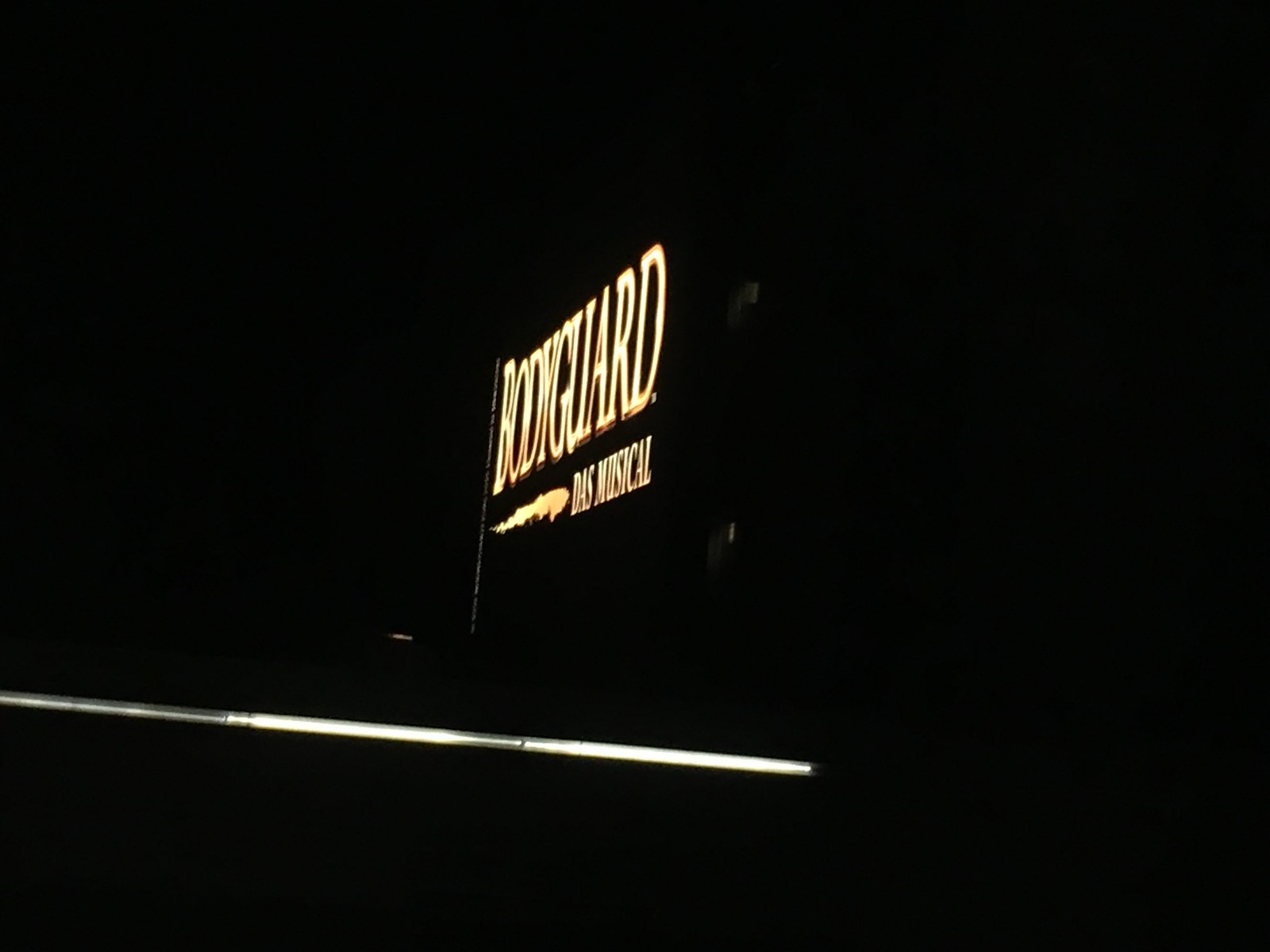This nighttime photo primarily features a brightly lit sign against a pitch-black sky. The sign, viewed from an unconventional side angle, reads "BODYGUARD" in illuminated white letters, with "Das Musical" written underneath in smaller text. There's a symbol between the texts that resembles a shark or an indistinct blob. The sign is attached to a structure, as indicated by a faint reflection of a pole supporting it. Below the sign, a long strip of fluorescent lights can be seen running along the eave of a nearby building, adding a subtle glow to the otherwise dark environment. The unconventional angle and low-quality of the photo make some details appear ambiguous, but the stark contrast between the lit sign and the surrounding darkness is clearly captured.